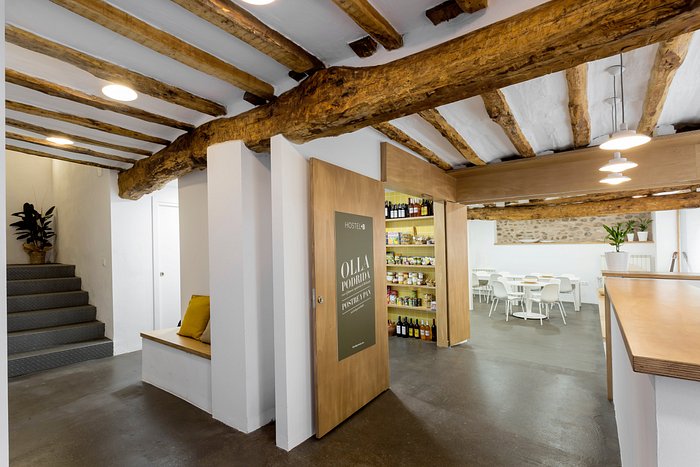The image depicts a basement-level restaurant or cafe with a cohesive blend of rustic and modern elements. On the far left, a set of gray steps leads down to the establishment's main area, where white plaster walls and ceilings contrast with exposed medium wood beams. Interspersed between the beams are recessed downlights that provide ample illumination. To the right of the staircase, there's a compact seating nook built into the wall, creating a cozy corner for patrons.

Directly in front of the entryway is a counter area topped with polished wood, complemented by old-style white pendant lamps hanging above. Adjacent to this is a pantry or display area featuring multiple shelves—colored yellow—stocked with wine bottles and other goods available for sale. The pantry's entrance, adorned with a sign that says "Ola," is flanked by a sliding door.

Further into the room, the dining area is visible, furnished with white tables and armless chairs arranged neatly. The decor includes white potted plants that add a touch of greenery to the space. The white walls are accented by a decorative horizontal stone feature, enhancing the room's aesthetic. Additionally, hints of natural light or additional lighting brighten the right side of the image, suggesting a well-lit, inviting atmosphere. The overall ambiance blends the warmth of wood with the sleekness of modern design, offering a welcoming and comfortable dining experience.